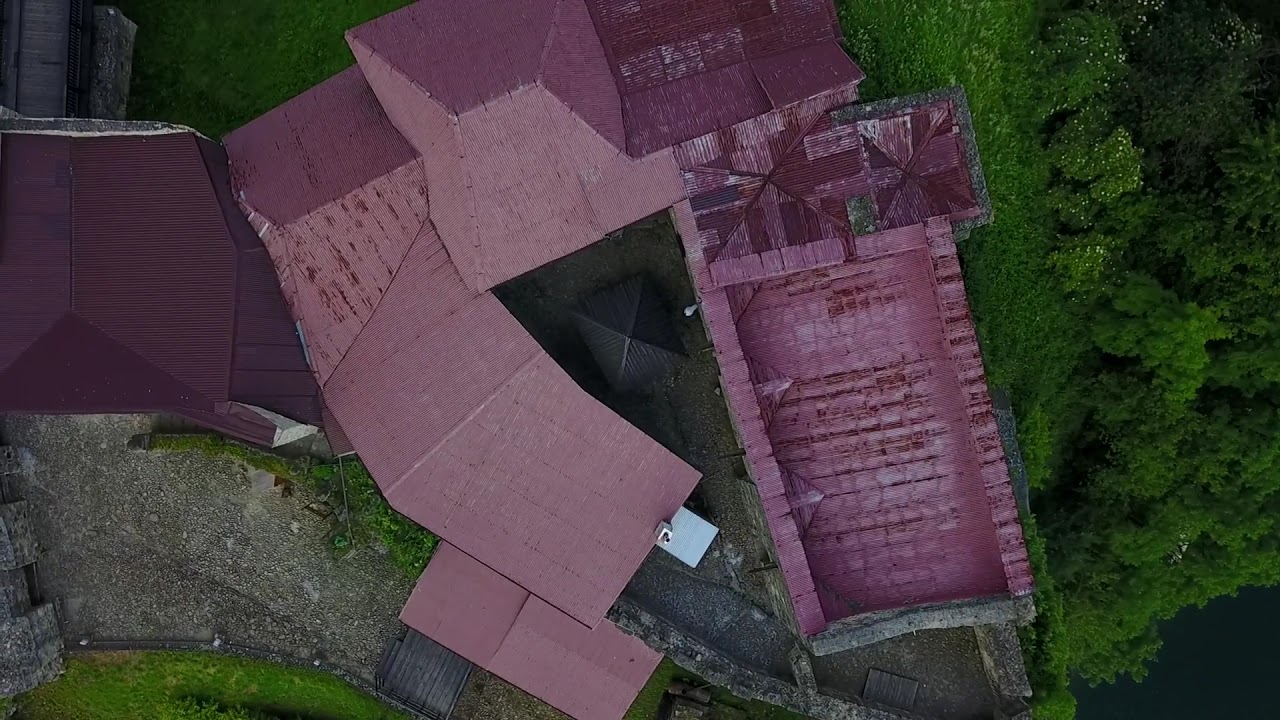This color photograph, taken from a drone, captures an aerial view of a sprawling, ancient-looking stone structure situated on a hillside. The building appears to be a historic monastery, castle, or villa, featuring a blend of old stonework interspersed with modern metal sheeting on various sections of the roof. These roofing sections include a main segment slightly left of center, extending downwards and curving to the right. The structure exhibits significant wear and tear, with moss growing over some stones, indicating its age.

The roof sections vary in condition, with some looking newer while others show more damage. The left side of the image features a paved road and a small wooden bridge, adding to the intricacy of the layout. On the right, the building borders a heavily forested area, with sloping turf leading downwards from the structure.

There’s a distinct open structure resembling an empty pool adjacent to the main building, colored dark red to match the roof. Surrounding the building are expanses of green grass and trees, contributing to the picturesque landscape. The photograph, measuring 8 by 5 inches, presents a detailed bird’s eye view without any people or text, capturing the essence of both ancient architecture and its natural surroundings.